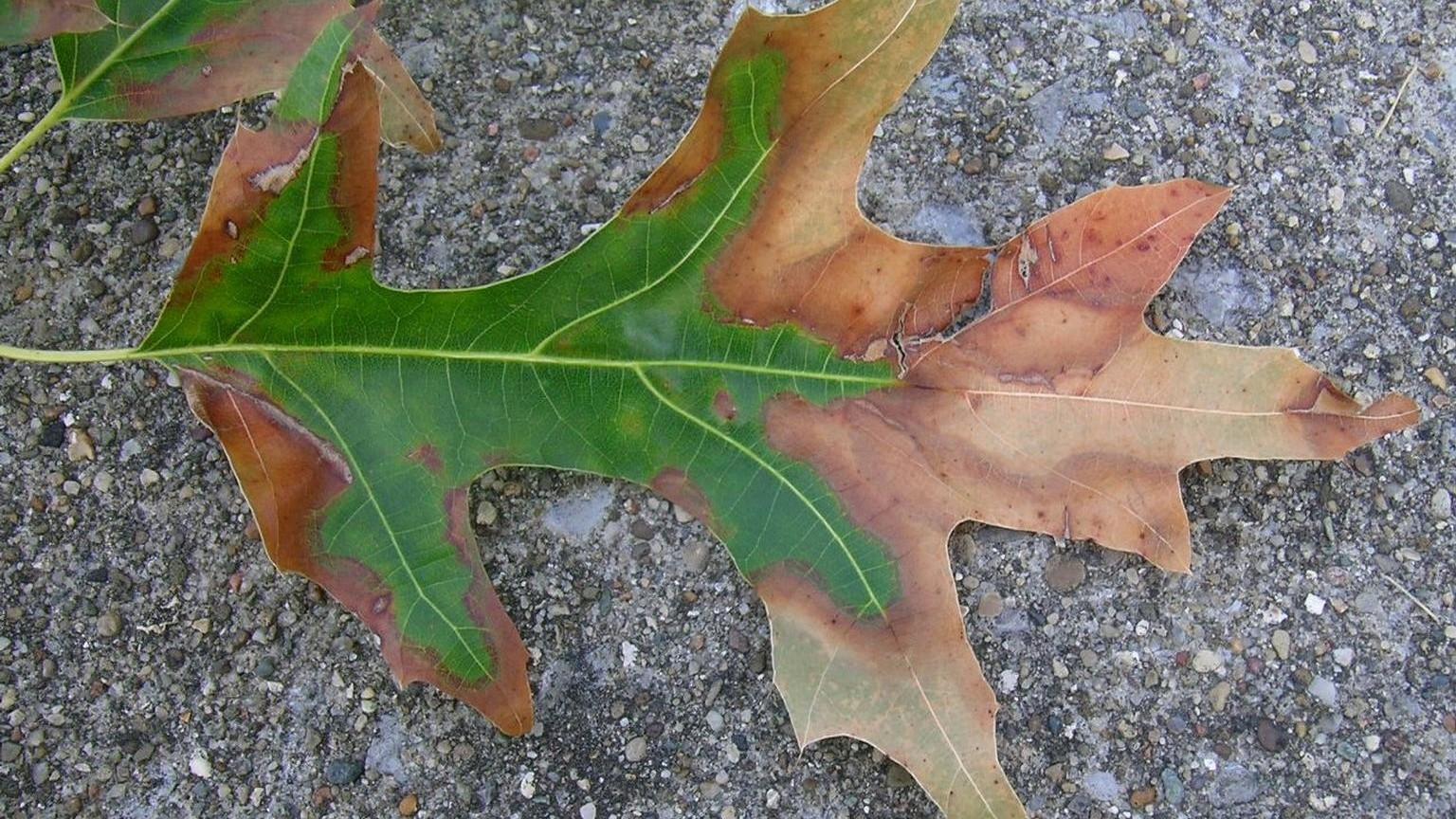In the image, two arched tree leaves are prominently displayed, one lying on top of the other on a ground scattered with small gray, black, and white gravels. The top leaf is green with a light green vein running along its center. It has a stretched-out stalk extending from the left side towards the center, with two smaller leaves on either side and a pointed tip. Below it lies a larger brown leaf, sharing a similar arched shape. The brown leaf contrasts with the vivid green leaf above, highlighting the transition from life to decay. The bottom leaf has a tear near its upper portion, adding texture to the scene. Both leaves have green stems and are positioned on an asphalt-like surface. The image dimensions resemble those of a wide high-definition television, emphasizing a broader, more panoramic view.